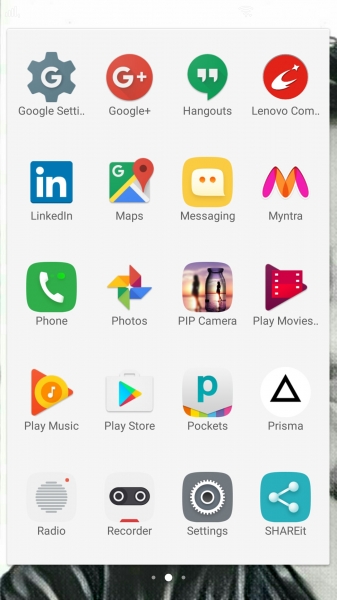The image displays a mobile phone screen brimming with various app icons on a black background. Starting from the top, we see the Google Settings icon followed by icons for Google Plus and Hangouts. There is a Lenovo app, a LinkedIn icon, and Google Maps prominently marked with a red pin. Next, a yellow square labeled "Mintra" beside an icon featuring purple legs with an orange center on either side.

Central to the display is a green square housing a white phone icon, representative of a calling app. Nearby, a photo gallery icon with a picture of a flower in a pinwheel design can be seen. There's also a PIP (Picture in Picture) camera app. The Google Play suite is represented by several icons: Play Movies with a sideways red triangle, Play Music with another sideways triangle, Play Store indicated by a briefcase-like icon with a play button.

Further down, the Pocket app is identifiable by a "P" with various colors—red, yellow, green, blue, purple, and pink—forming a background. The Prismo app is marked by a triangle consisting of merged colors. The Radio feature is depicted onscreen with a traditional radio icon and a speaker symbol, red in the top right corner. The Recorder app appears blue with dots inside, followed by a generic black square and gray square icon.

In proximity lies the Settings icon, followed closely by a "Share it" application. The background behind all these icons is a solid black, ensuring that each app symbol stands out clearly.